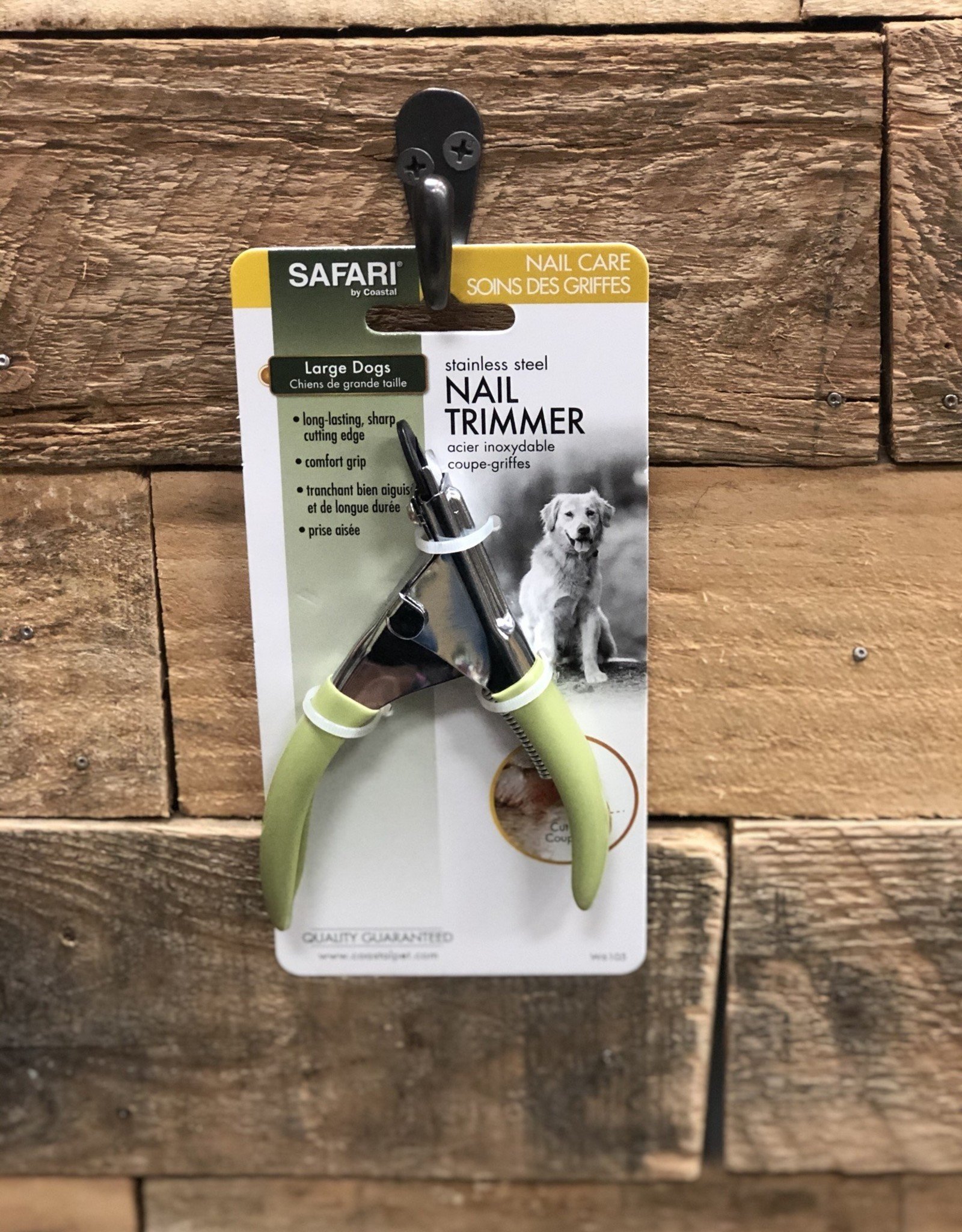The image depicts a package of Safari nail trimmers for large dogs, hanging on a black hook mounted with two screws on a light-colored, wooden slatted wall. The trimmers, featuring silver blades and pale green handles, are secured in white cardboard packaging, which is further held together by zip ties. Branding and product information dominate the packaging, with an olive green strip at the top reading "Safari." Below, the text specifies that the trimmers are designed for large dogs, highlighting attributes such as long-lasting sharp cutting edge, comfort grip, and stainless steel material. Additional details repeated in a different language, likely French, mirror these key features. An image of a dog, resembling a golden retriever, is visible on the right side of the packaging. The setting appears to be either a home or a store displaying the product.